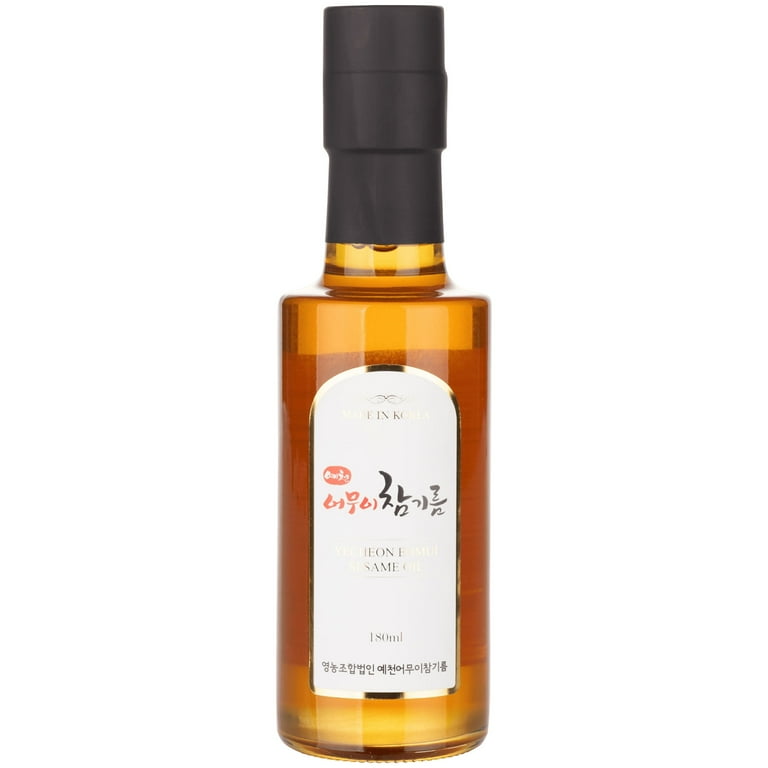The image features a glass bottle, prominently displayed against a white background. The bottle contains a liquid of varying amber hues, from light to deep dark amber. Featuring a long neck sealed with black plastic wrapping, it stands upright and slender. The label on the bottle is white with black and red writing, written in Korean characters, albeit mistaken for Japanese by some. The single focal point is the product itself, an 180-milliliter bottle. The label’s top and bottom are curved, with additional details including a mix of peach and black text. The visible English letters on the label include sequences like "E-O-N" on the upper part and "S-A-M-E" on the lower part, although some are faded. The glass body of the bottle appears to have a faceted shape, enhancing its elegance.